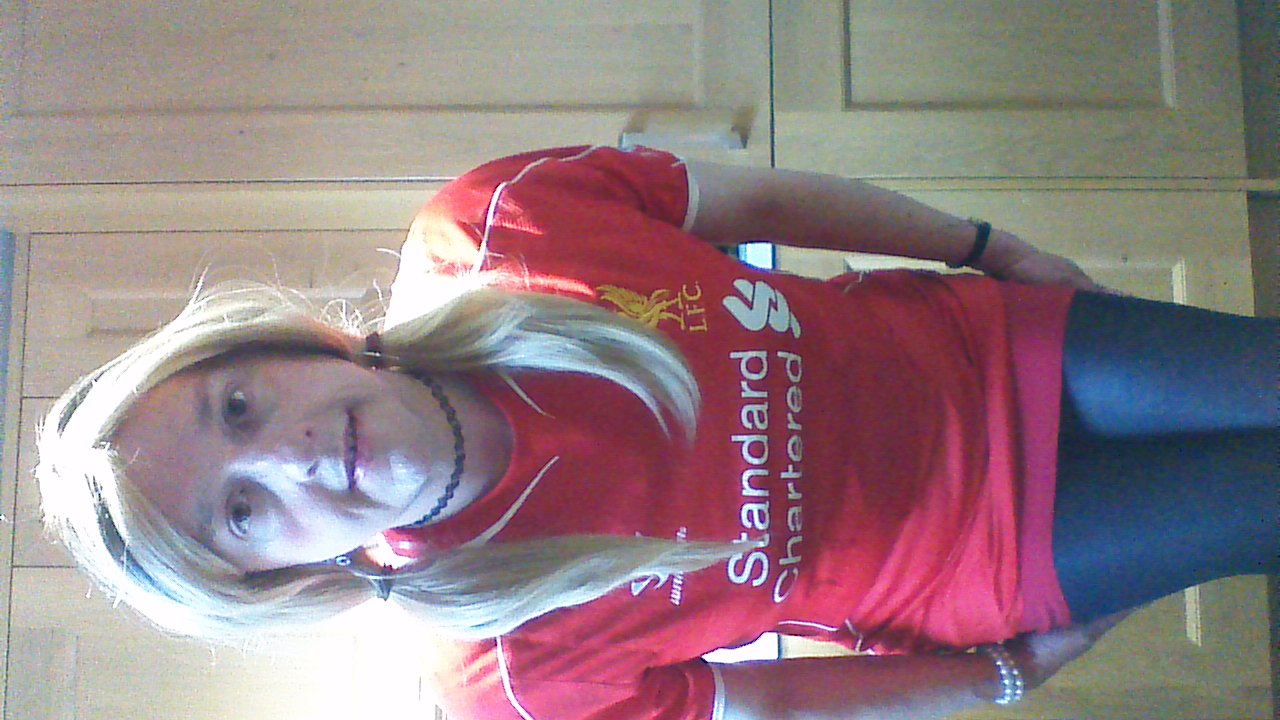The image depicts a person with a distinctly masculine appearance posing indoors, against a backdrop of closed wooden cabinet doors. They are dressed in a red sports jersey emblazoned with "Standard Chartered" and the "LFC" logo featuring a golden griffin, paired with blue skinny jeans. The individual, likely of Caucasian descent, has a blonde wig styled into pigtails that cascade over their shoulders. They are wearing a lace choker around their neck, pink lipstick, and have no visible eye makeup. They also display some jewelry: a double-beaded pearl bracelet on one wrist and a black watch on the other. The person seems a bit awkward, bending slightly at the waist as if to fit into the frame, with their hands resting on the back of their thighs, and they are offering a slight, somewhat forced smile, revealing a bit of their teeth. The overall appearance suggests they might be in their 40s.